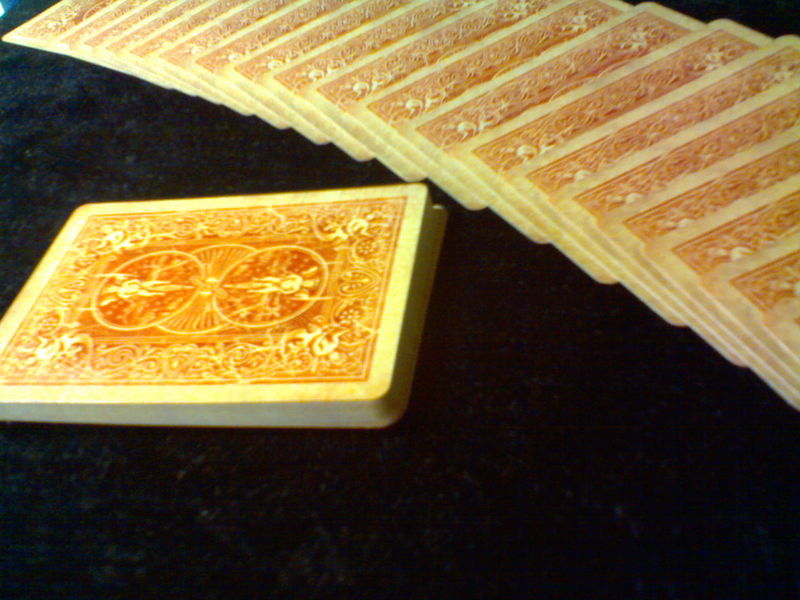In the photograph, a set of playing cards is artfully arranged on a dark marble surface, showcasing intricate details. The black marble tabletop exhibits faint gray veining, adding a touch of elegance to the background. At the center left of the image, a neatly stacked deck of playing cards displays their detailed orangey-red patterned backs, which feature what appear to be light red or orange markings, possibly suggesting wear or an intentional design. To the right of the image, a series of cards are fanned out in a graceful curve, extending from the center towards the top left, laying on top of each other and creating a visually dynamic composition. The photograph captures the texture and intricate beauty of both the playing cards and the sophisticated marble surface.